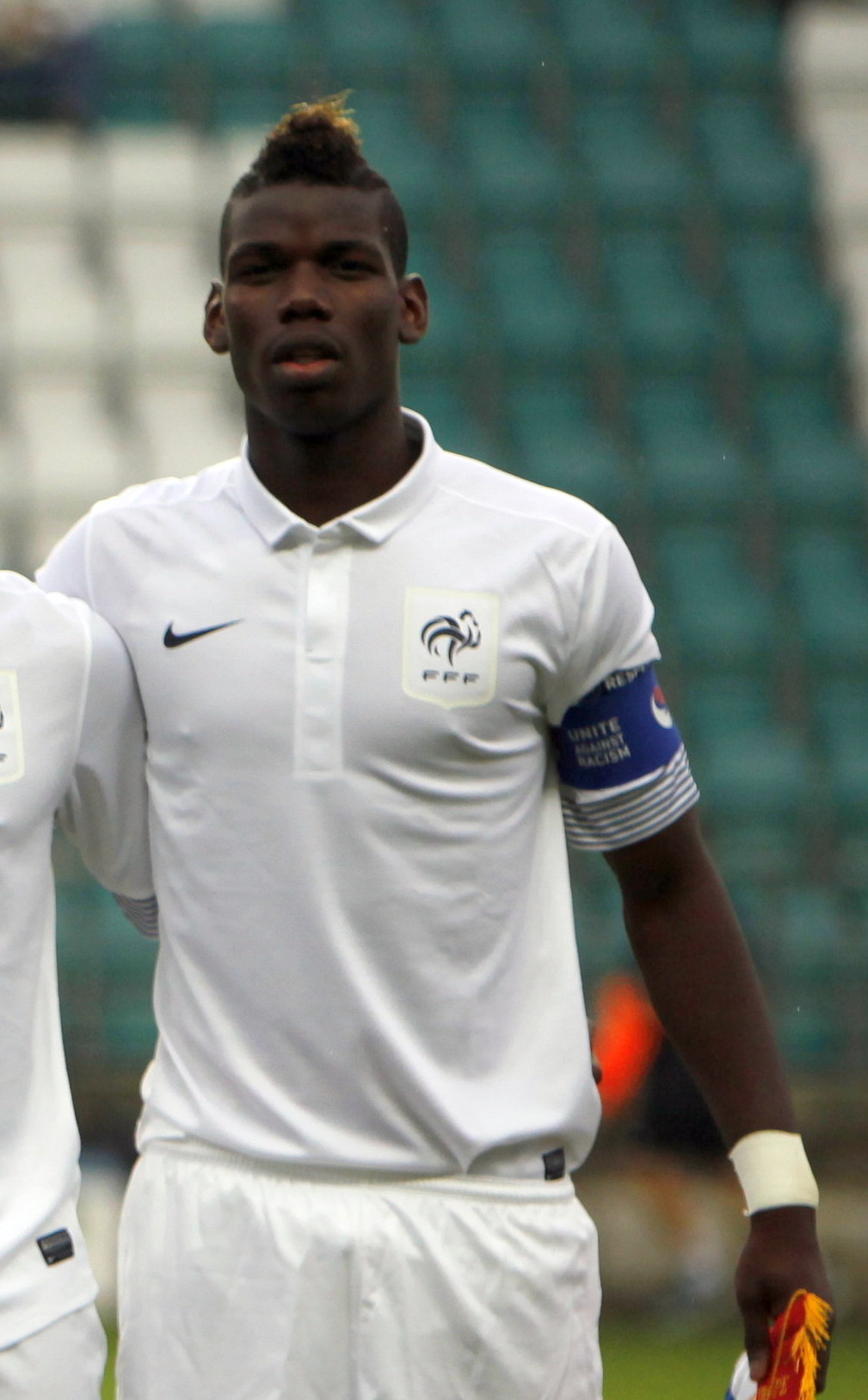In the image, there is a young African-American man, likely in his early 20s, standing on a field with stadium seating visible behind him. The seats appear to be white and green, arranged in rows but unoccupied, suggesting a practice session. The man has dark skin and sports a distinctive short mohawk with the top dyed blonde. He is wearing a white, short-sleeve t-shirt featuring a Nike logo on the left chest and an FFF crest on the right breast. Additionally, he has a blue armband on his upper bicep that reads "Unite Against Racism." Around his right wrist is a white wristband. The man is squinting with his mouth open, and his arm is draped around another person on the left edge of the photo, though only the shoulder of this second person is visible.